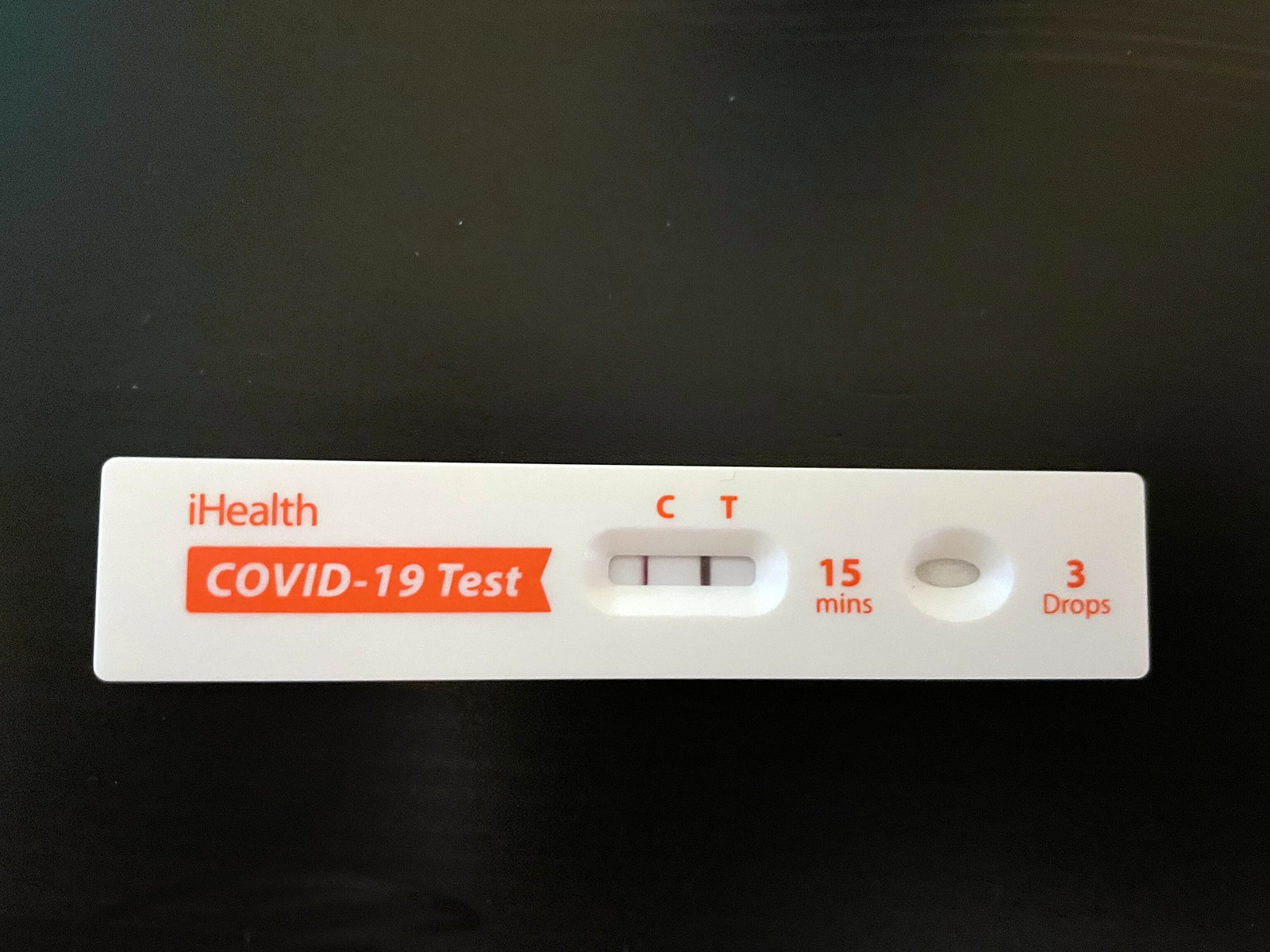In this image, we see a COVID-19 home test kit displayed prominently. The background is a gradient transitioning from greenish-gray at the top to black at the bottom and is intentionally blurred to keep the focus on the test. The test itself is white and rectangular. At the top of the test, the brand name "iHealth" is written in red. Just below the brand name, there is a red ribbon-like strip with the text "COVID-19 Test" printed in white.

In the center of the test strip, there is an oval-shaped window showing two lines: one is dark black and the other is a lighter black or red line. Above this window, the letters "C" and "T" are present, indicating the control and test lines, respectively. Beneath the oval window, "15 MINS" is written to denote the 15-minute testing time.

Additionally, there is another small oval shape encircled in white, next to which the number "3" is displayed in bold red. The word "DROPS" is printed in red beside this circle, indicating the number of drops of the sample required. 

The design and simple instructions on the test make it clear and easy to understand.